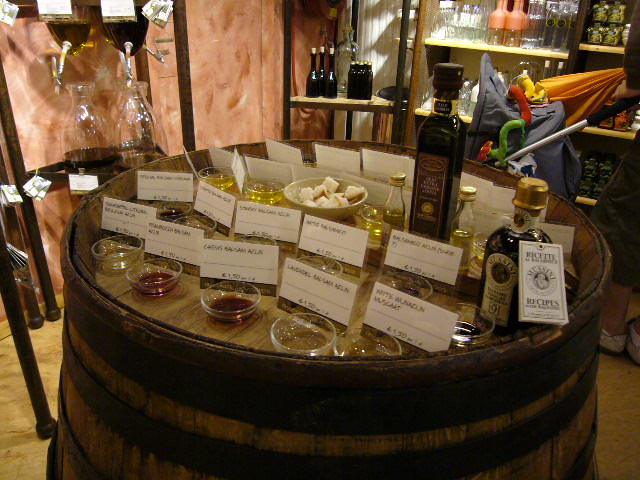The indoor photo appears to be taken at a specialty store, possibly a wine shop or a gourmet store, focused on sampling. At the center of the image is an old wine barrel serving as a sampling table, topped with various bowls containing different liquids—some clear, some yellow, and some red. Each bowl has a sign in front of it, though the writing is slightly blurry. A bowl of bread is also present, suggesting the liquids could be oils or vinegars rather than liquor. Surrounding the barrel are several glass bottles, including one large bottle and smaller ones, placed next to the bowls. The background features shelves stocked with additional bottles and glasses. To the left, there’s a dispenser system that might be filling large glass containers. Meanwhile, on the right side of the image, a person with a baby stroller, adorned with hanging toys, is visible, further illustrating the vibrant setting of the store.